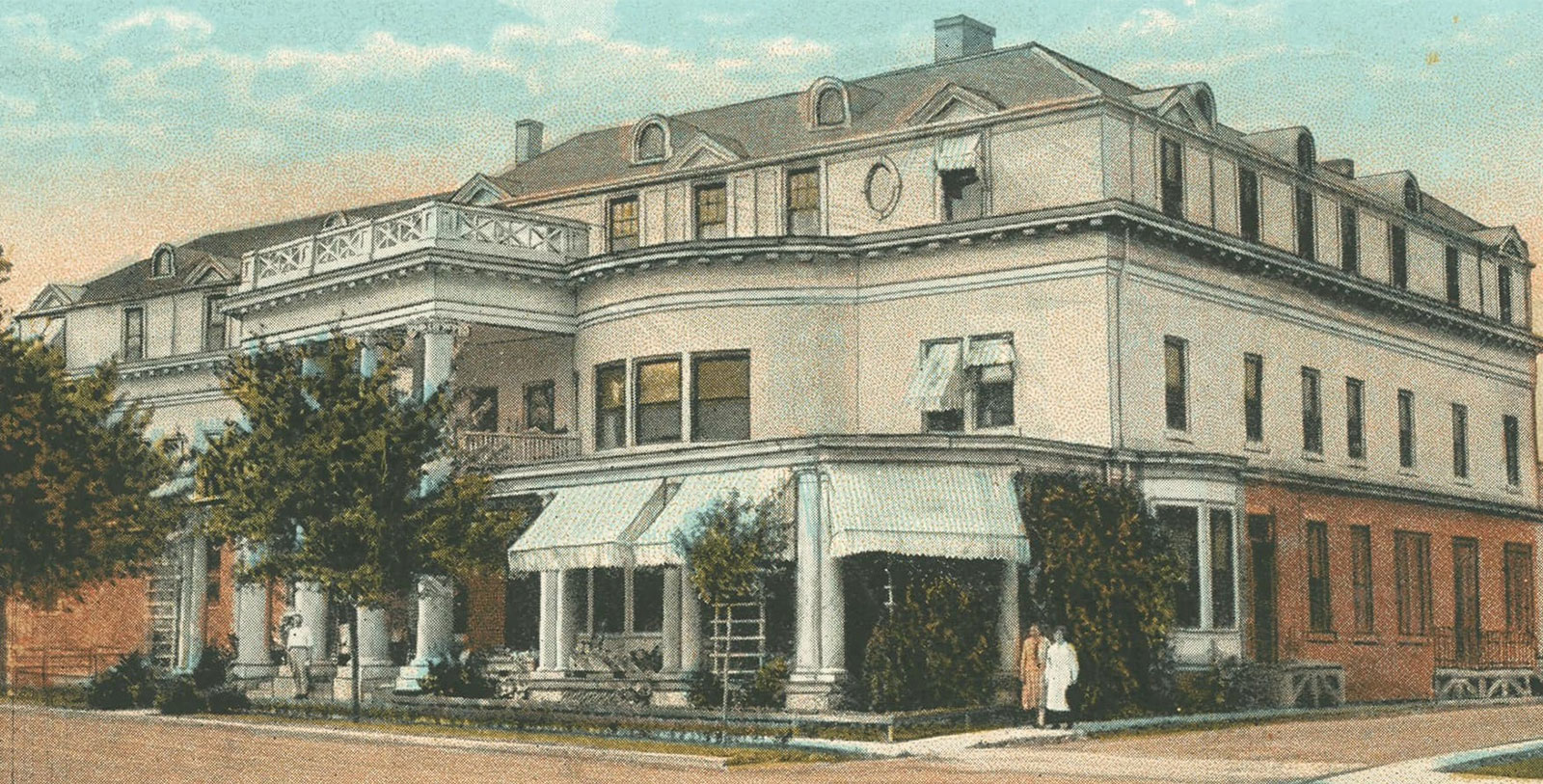The image is a detailed artist's rendition of a grand, three-story building, likely from an era over a century ago, exuding a postcard-like charm. The structure, possibly a lavish mansion or significant residential building, occupies roughly half a city block and is reminiscent of Georgian architectural style with elegant elements akin to the U.S. White House. 

The building's first floor features red brick, while the upper floors are a smooth stone color or white plaster. Tall colonial columns support an awning at the entrance, leading up to a third-floor balcony, flanked by dormer windows and multiple chimneys. The roof appears to be covered in an expensive granite-like material.

Along the front and sides of the building run brick-colored sidewalks bordered by lush shrubbery and trees. The ground level also includes what was likely an open porch now enclosed, adorned with a bay window. In the vicinity, trellises with climbing plants add to the pastoral aesthetic. Two figures in old-fashioned attire can be seen walking towards the front of the building, almost giving a sense of motion and life to the scene.